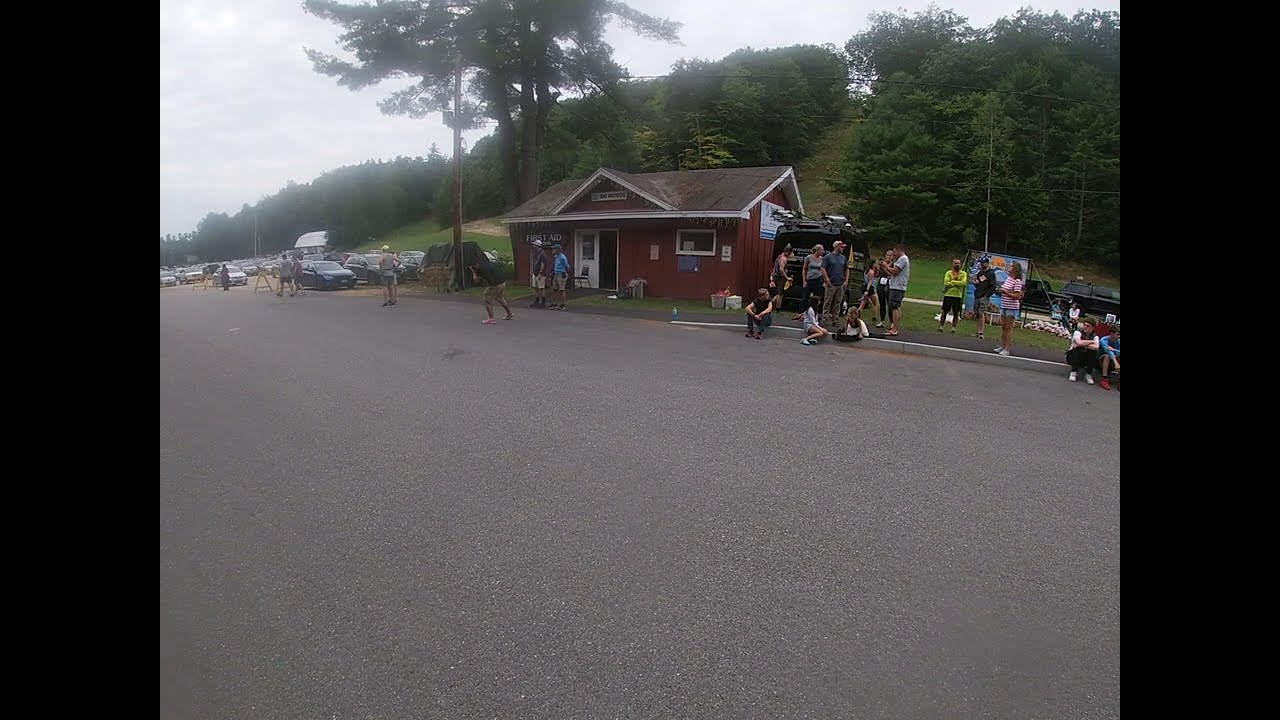The photograph showcases a broad, empty asphalt street dominating the lower portion, bordered by minimal sidewalks and curbs where several people are positioned either sitting or standing. In the center background, there is a small red building with a black roof and white accents, possibly a concession stand or shop, featuring a white door adorned with unreadable signs. Adjacent to the building on the right, a black van is parked, with nine individuals nearby, three seated and others standing. One man in different colored shoes leans down, seemingly taking a picture. On the left side, a dirt patch parking lot is filled with numerous cars. In front, various groups of people are scattered, with some on the curb and others in the grassy area. Further back, a lush, green hill rises, densely populated with tall, leafy trees, and a dirt path extends into the wooded backdrop. The entire scene suggests a gathering, perhaps in anticipation of a parade or event.